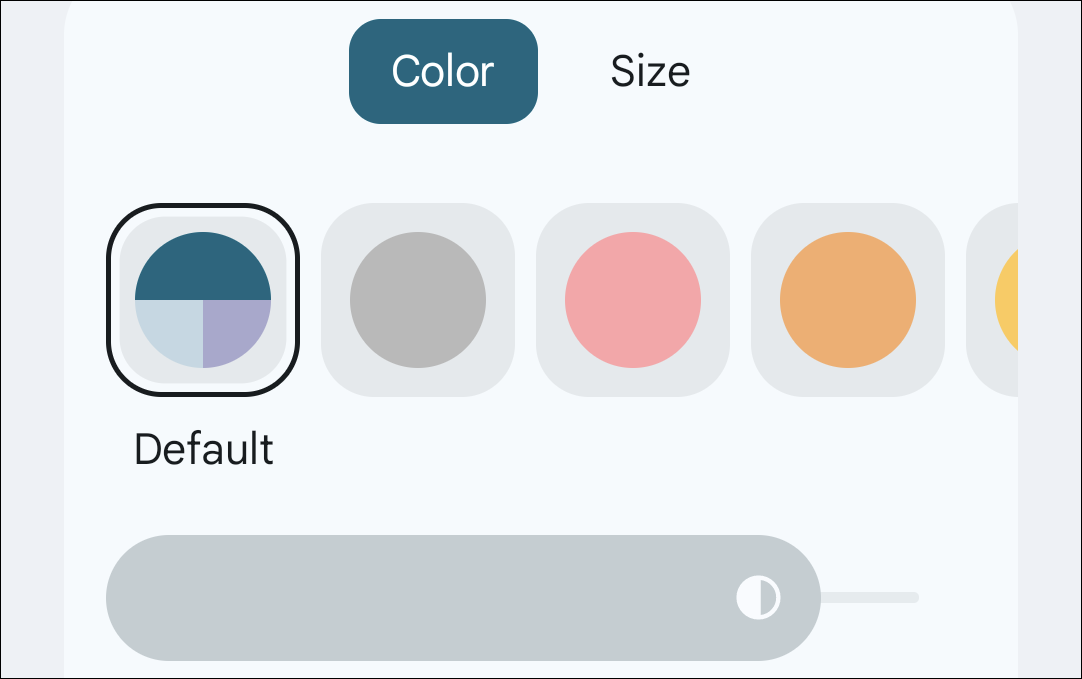The screenshot primarily showcases a user interface on a white background. At the top, a bluish-green button with white text reads "Color." To its right, the word "Size" is displayed in black font. Below these labels are four rounded square options, with the first one outlined in black to indicate selection. 

1. The first option, labeled "Default," contains a circle segmented into three colors: the top half is bluish-green, the bottom left is light blue, and the bottom right is purple.
2. The second option features a solid gray circle.
3. The third option includes a pink circle.
4. The fourth option contains an orange circle.
5. There is a partial view of a fifth option, which shows a yellow circle.

Below these options, there is a large gray field, possibly a search field. On the far right of this field is a circle divided into two halves: the left half is yellow, and the right half is gray. This concludes the main elements visible in the screenshot.